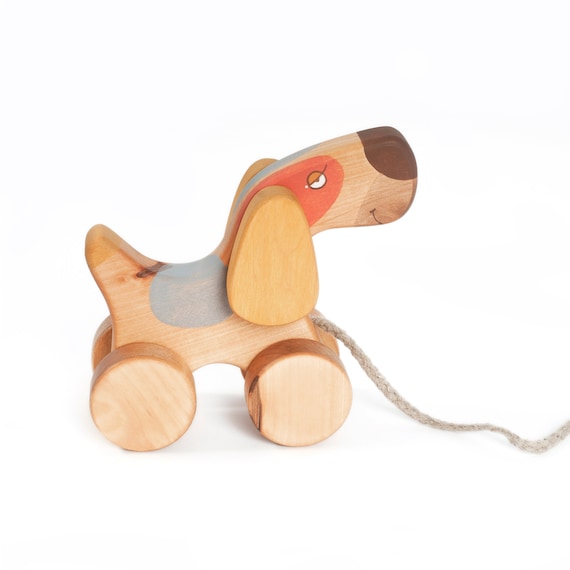This photograph showcases a charming child's toy: a meticulously carved wooden dog. Ingeniously designed with round wheels in place of feet, the dog can be easily pulled along by a child using the attached braided cotton rope. The toy exhibits the natural beauty of its light-colored wooden finish, complemented by delightful painted accents. The tip of the dog's nose is painted a warm brown, while a splash of coral pink adorns the area around its eye. Adding a touch of character, a gray spot is painted on the dog's back. The white braided cotton rope enhances the toy's playful yet simplistic aesthetic, making it an adorable and functional keepsake for any child.